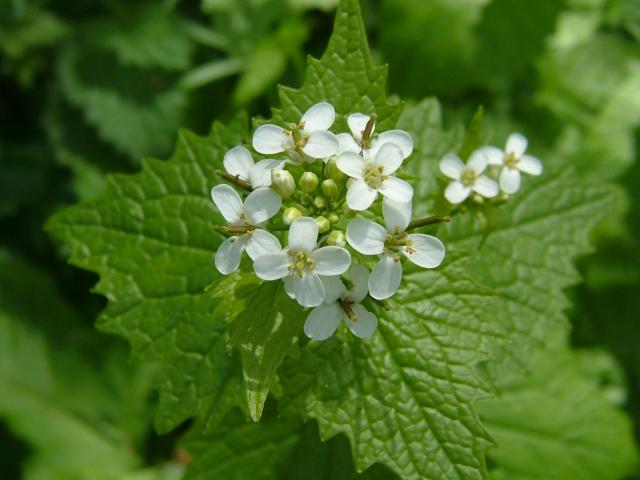This close-up photograph captures a top-down view of a flowering plant, showcasing a central cluster of delicate white flowers. Each flower features a very pale green center and four elongated, half-circle petals arranged symmetrically—two at the top and two at the bottom. Surrounding the flowers are vibrant green leaves with pointed tips and prominently visible veins, adding a striking contrast to the soft white blossoms. In the very center of the floral cluster, several unopened buds stand out, cylindrical in shape with light green hues blending into their unopened petals. The background fades into a blurred tapestry of green leaves, highlighting the intricate details of the flowers and leaves in the foreground.